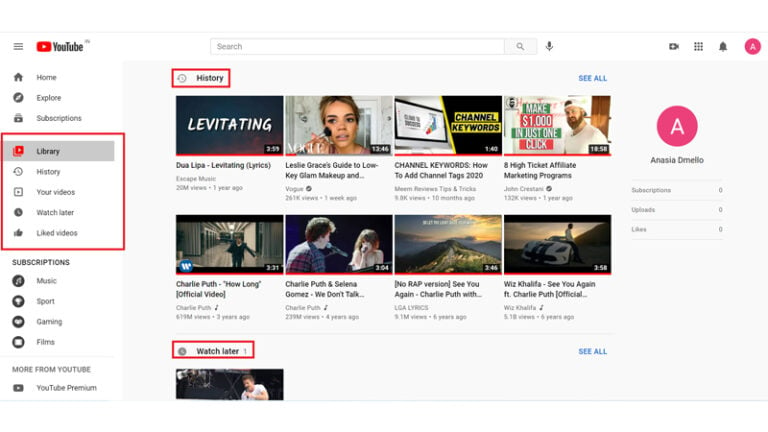The image depicts a YouTube page with a standard white background. Specific parts of the interface are highlighted with red boxes, suggesting a focus for educational purposes. The top left corner features the familiar three-bar menu icon, next to which is the YouTube logo—a red rectangle with a white play arrow and the word "YouTube" in black.

Directly beneath the logo, the sidebar menu lists several options: Home, Explore, Subscriptions, Library, History, Your Videos, Watch Later, Liked Videos, Subscriptions, Music, Sports, Gaming, Films, and More from YouTube including YouTube Premium. The entries Library, History, Your Videos, Watch Later, and Liked Videos are encased in a red box, implying their importance.

To the right of the sidebar, the main content displays the "History" section. Under the "History" header, there are eight video thumbnails organized in two rows of four. Each row is framed with a red box, drawing attention to these specific videos. The videos in the first row include:

1. "Dua Lipa - Levitating (Lyrics)"
2. "Leslie Grace's Guide to Low-Key Glam Makeup"
3. "Channel Keywords: How to Add Channel Tags (2020)"
4. "Eight High-Ticket Affiliate Marketing Programs"

Just below "History", there's a "Watch Later" section with one visible video. This section is similarly encased in a red box.

Overall, the red boxes highlight sections likely intended for a tutorial or instructional guidance on how to navigate or utilize features within the YouTube platform.